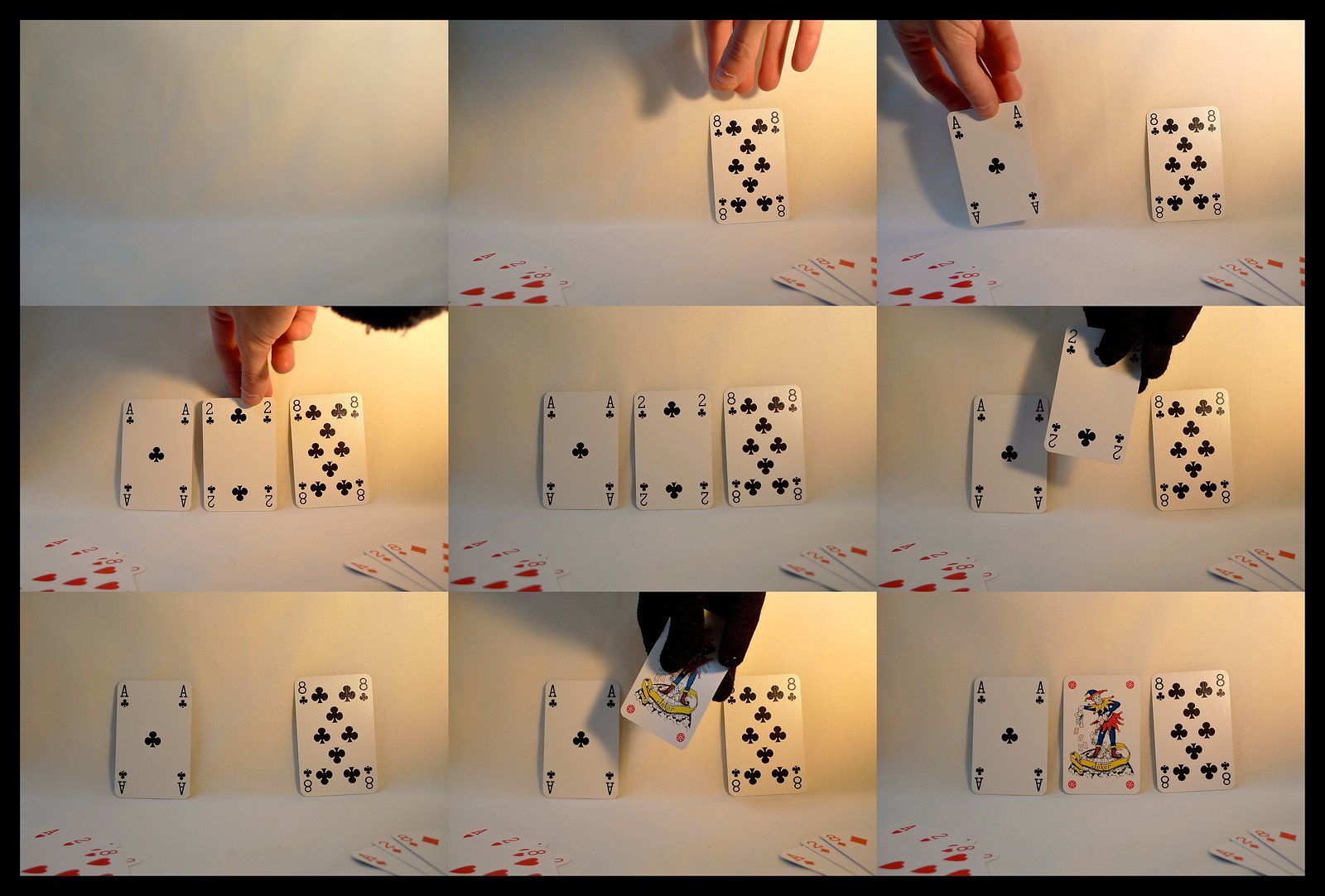The image sequence showcases a step-by-step progression of a card trick, divided into nine sections, each portraying different stages of the trick with various angles. 

1. The first section displays an Eight of Clubs against the backdrop of a wall.
2. The second section shows an Ace of Clubs positioned almost adjacent to the Eight.
3. In the third section, a Two of Clubs is placed in between the Ace and the Eight.
4. The fourth section mirrors the third but without a hand in the frame.
5. The fifth section captures the moment where a gloved hand (wearing a black glove) is about to remove the Two of Clubs.
6. The sixth section displays only the Ace of Clubs and the Eight of Clubs, with the Two of Clubs completely removed.
7. The seventh section introduces a Joker, seemingly about to be placed in the gap between the Ace and the Eight.
8. The eighth section continues to suggest the Joker's placement, now partially hovering between the other two cards.
9. The final section depicts the Ace of Clubs, the Joker in the middle, and the Eight of Clubs, with no hand present, signifying the completion of the transition of inserting and replacing the middle card.

This series likely demonstrates a card trick, revealing the methodical process of removing one card and seamlessly substituting it with another.